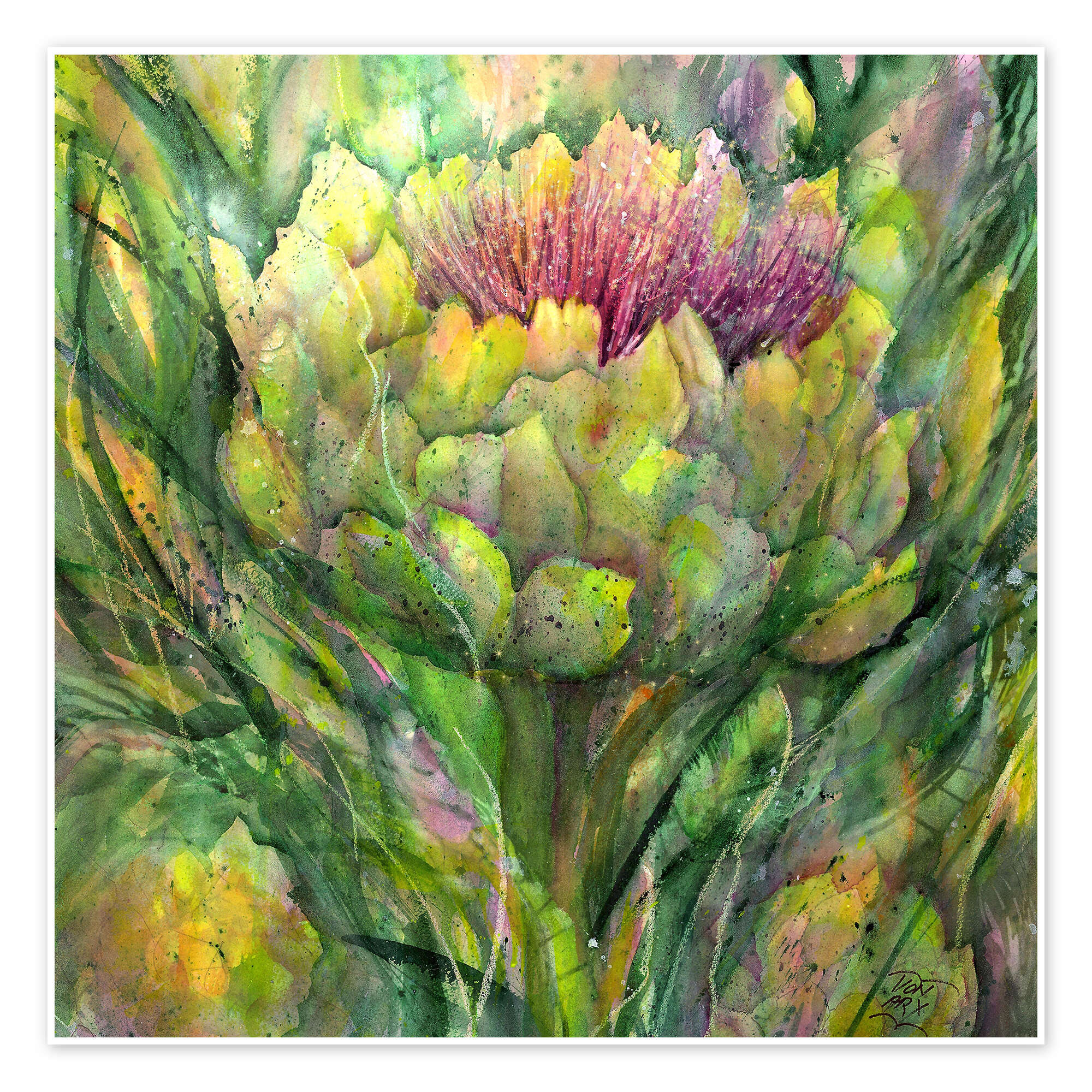This is a highly detailed watercolor painting, predominantly rendered in shades of green with accents of light amber and pale yellow. The composition, which fills the entire canvas without any white space, depicts what appears to be a thistle plant. The image is abstract yet clearly portrays a central flower with multiple petals and distinctive features. The painting shows a giant seed head at the plant’s center, from which pink, needle-like pollen threads emerge, enhancing its resemblance to a thistle. Layers of color blend seamlessly in a characteristic watercolor style, with darker hues overlaying lighter ones. The petals and leaves create a sense of upward movement through the use of varying greens and yellows, while streaks of white, possibly added with another medium like white charcoal or colored pencil, suggest texture and depth. Yellow circles peppered throughout may represent additional budding flowers. The painting is signed "Vaughan Arcs" at the bottom in marker.